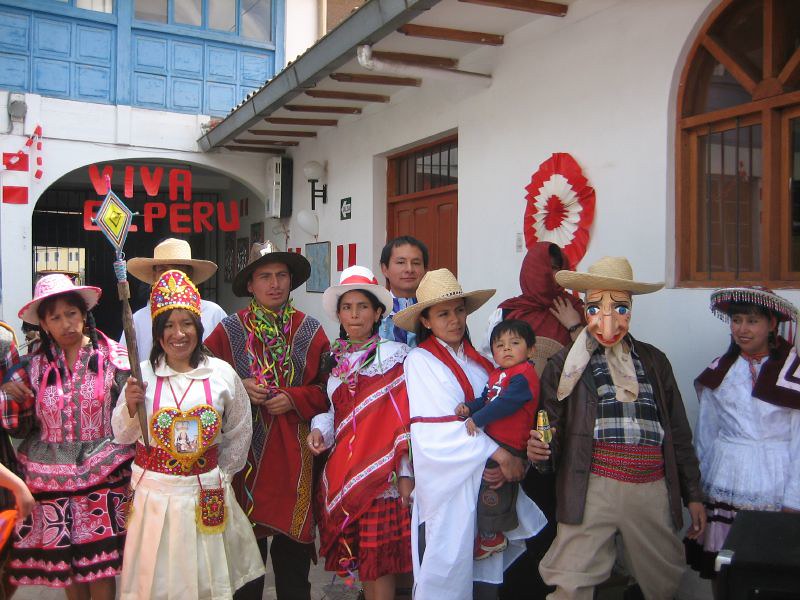In this captivating outdoor photograph, a lively group of people is depicted in traditional celebratory attire, reminiscent of classical Mexican or Latin American influences, possibly Aztec or Mayan. The scene is set on a stone or concrete brick ground, with a picturesque building in the background. Dominating the left side, a woman wears a striking white dress paired with an elaborate red and yellow headdress that evokes the grandeur of a pope's mitre. She holds a wooden staff adorned with a metal-capped jewel, adding a touch of mysticism to her appearance. On the right side, an individual dons a caricature mask, enriching the festive vibe. Additional members of the group wear a mix of sombreros and cowboy-style hats, all dressed in vivid, celebratory outfits that splash colors such as red, white, blue, maroon, green, pink, purple, and gray across the scene. Central to the composition is a large banner emblazoned with the partially visible text "Viva El Peru," hinting at a festive celebration in Peru, all bathed in the bright light of midday. The crowd's collective gaze directs towards the camera, establishing a stark visual connection with the viewer and grounding the lively atmosphere in a specific cultural and geographic setting.